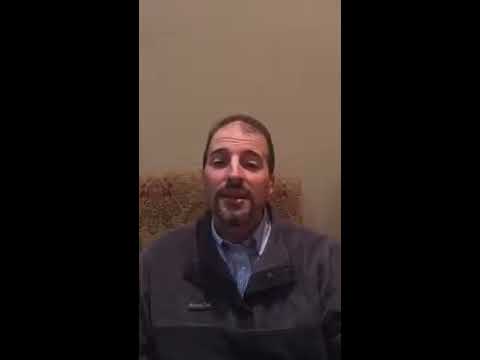This is a vertically oriented portrait of a white male with balding, thin dark brown hair, and prominent dark brown eyebrows. He has a distinctive thick dark brown circular goatee and mustache that link together around his mouth and chin. He is dressed in a blue button-down collared shirt, layered with a dark gray and black striped fleece pullover that is unzipped at the neck. The setting appears to be a video scene, with the man facing the camera and seemingly in conversation. The background features a white wall with a shaggy rug or a similar textured square object placed in front of it. The image quality is low, marred by significant compression artifacts, and displays two solid black rectangles on each side, framing the portrait.